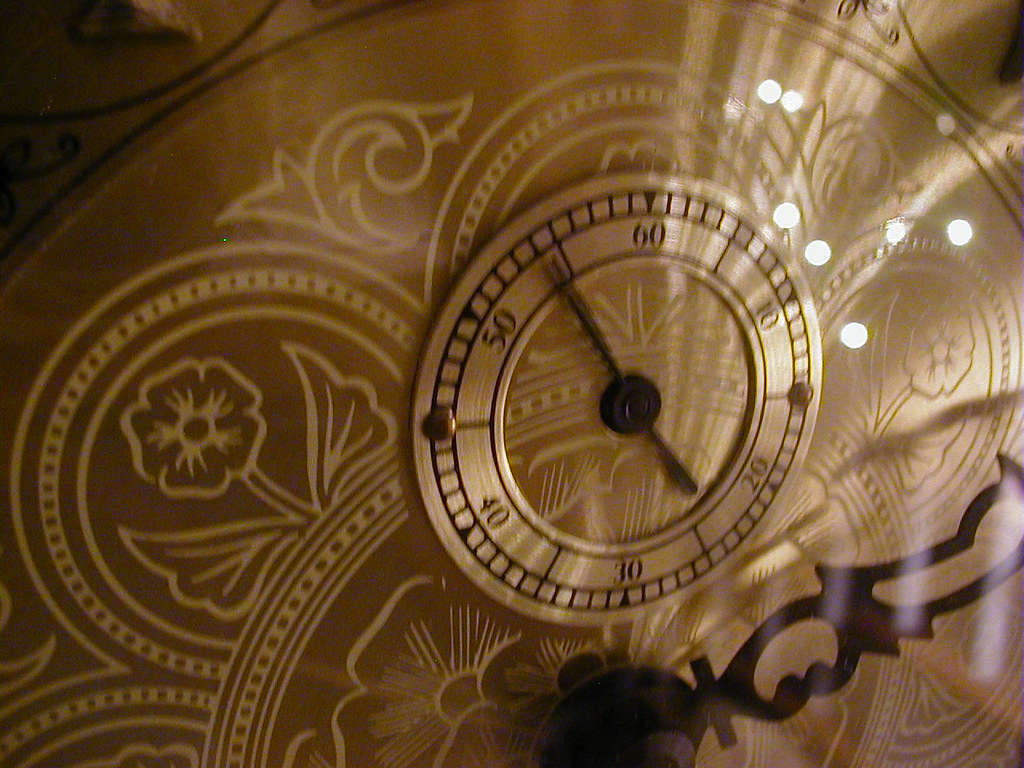This image depicts the intricate face of a circular, golden clock. Encircling the clock are numerals marking the minutes: starting with 60 at the top, followed by intervals of 10, 20, 30, 40, and 50, all arranged in a clockwise direction with smaller tick marks marking the individual minutes in between. At the center, a black hand is mounted on a black circular gear, indicating the passage of time in seconds. The golden face of the clock is adorned with delicate, white floral symbols, adding an ornate and elegant touch to its overall design.